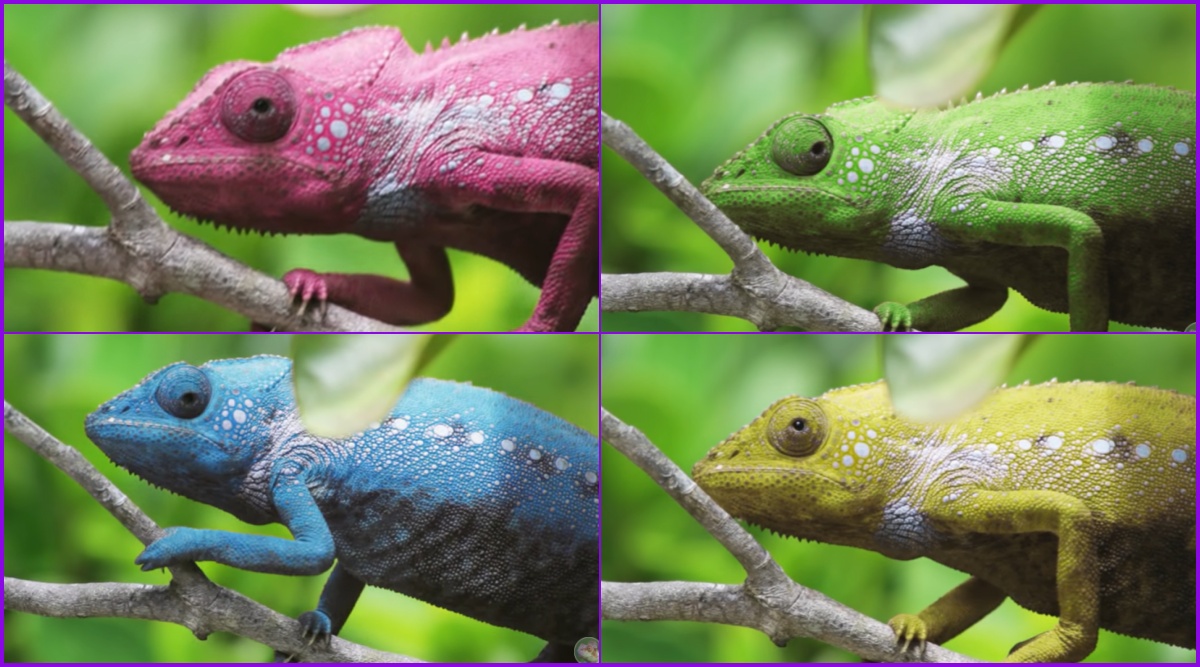The image is divided into four sections, each displaying a chameleon in different colors and postures, suggesting various moments or angles. The top left section shows a pink chameleon in close-up, adorned with tiny white circles and slash-like marks, its eye centered. In the top right, the chameleon appears green with its eye shifted rightward. The bottom left features a blue chameleon looking slightly downward, climbing a branch partially covered by a leaf near its neck. Lastly, the bottom right section depicts a yellow chameleon with its eye centered, looking up. Like the other segments, this chameleon also has a leaf partially covering its neck. The chameleons, showing an array of pastel colors and white brush-like speckles, seem digitized, adding a surreal quality. Positioned on a bright tree branch, their limbs are outstretched, indicating movement despite their seemingly calm demeanor.